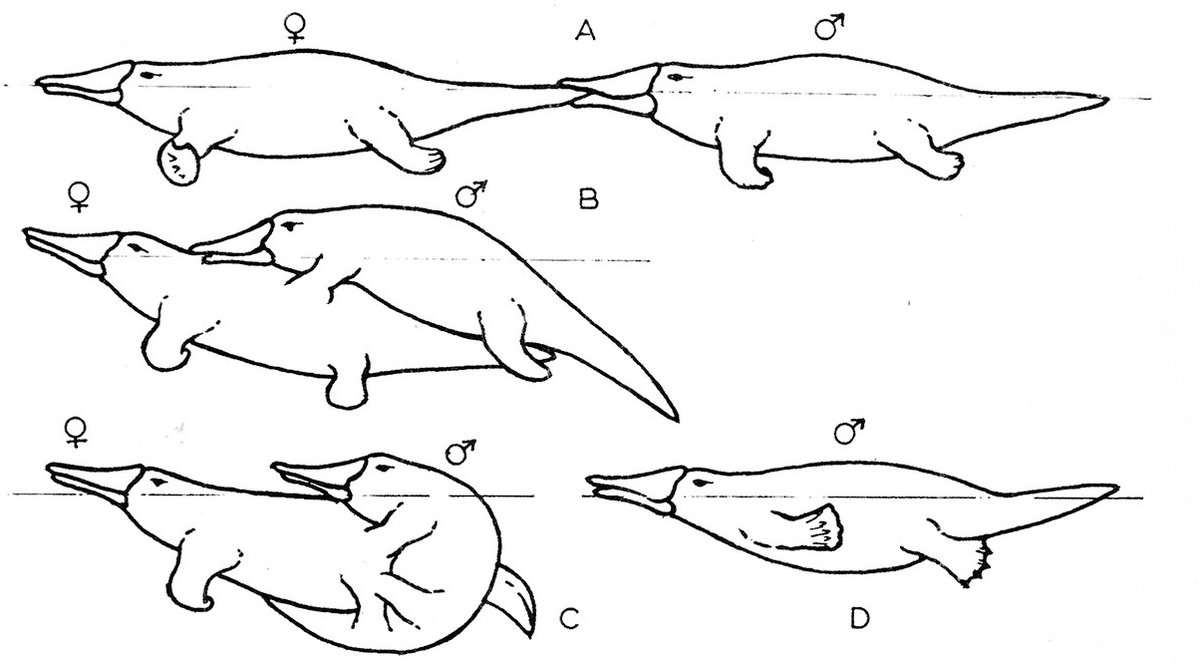The illustration consists of a sequence of four black-and-white drawings labeled A, B, C, and D, depicting the mating process of platypuses. In the first image (A), a female platypus swims horizontally leftward while a male platypus bites her tail with his beak. Both platypuses are denoted by circular symbols indicating their genders. The second image (B) shows the male platypus mounting the slanted-up female from behind. In image C, the male appears to wrap around the underside of the female in a reverse C-shape. Finally, in image D, the male platypus is seen swimming alone horizontally, looking visibly different or possibly unhappy, with no female present. This sequence seems to illustrate the progression of platypus mating behaviors.